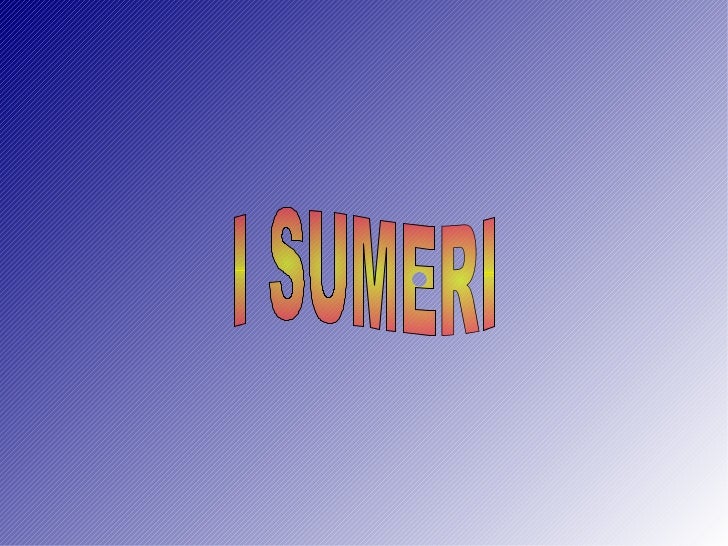The image features a gradient background transitioning diagonally from a dark blue in the upper left corner to almost completely white in the bottom right corner. This gradient exhibits a subtle line pattern throughout, contributing to a textured appearance. Centrally positioned in the image is large, bold text with a black outline, spelling out "I SUMMARY" or possibly "I SUMERI" depending on interpretation. Each letter of the text showcases its own gradient that transitions from dark red at the top, through yellow in the middle, to dark red again at the bottom. Notably, the letter "E" has a distinctive hole in the middle, revealing the background pattern behind it. The overall aesthetic of the image suggests it might have been created using an old Windows application like Microsoft Paint or Windows Movie Maker, and there is a slight static overlay that gives it a retro digital feel.